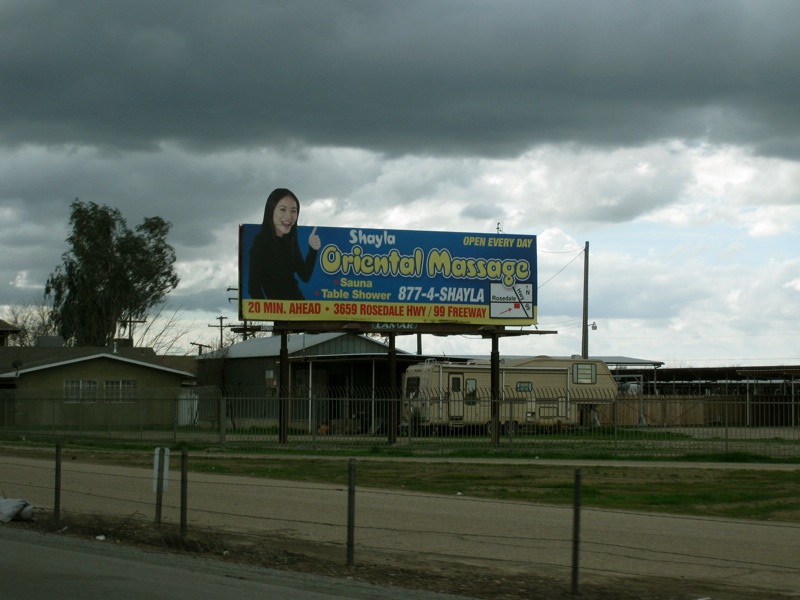Beneath a stormy sky heavy with dark bluish-gray clouds, a partially illuminated photograph captures a scene during the day. The left side of the image features a chain-link fence running parallel to a light gray asphalt road marred with darker patches from repairs. Adjacent to the road is a large patch of grass showing signs of sunburn, with sections of dark green, yellow, and light brown.

Dominating the center of the image is an elevated, color billboard towering over the scene. The billboard advertises "Shyla's Oriental Massage" in bold white letters, with additional information like "Open Every Day," "Sauna," and "Table Shower" also prominently displayed. The featured image on the billboard depicts an Asian woman with straight black hair, a big smile, and a dark blue long-sleeve shirt, holding a thumb up. The contact number, "877-4-SHYLA," is visible, and below it, a yellow rectangle with red text reads, "20 minutes ahead," followed by the address "3659 Rosedale Highway / 99 Freeway."

Beneath the billboard, there's a beige RV with multiple windows and a tan door outlined in dark chocolate brown. Nearby are several buildings in various shades, including chocolate brown and gray, some with rope details. The scene is completed by a large section of light brown fencing, giving the impression of an urban landscape transitioning into a more commercial zone.